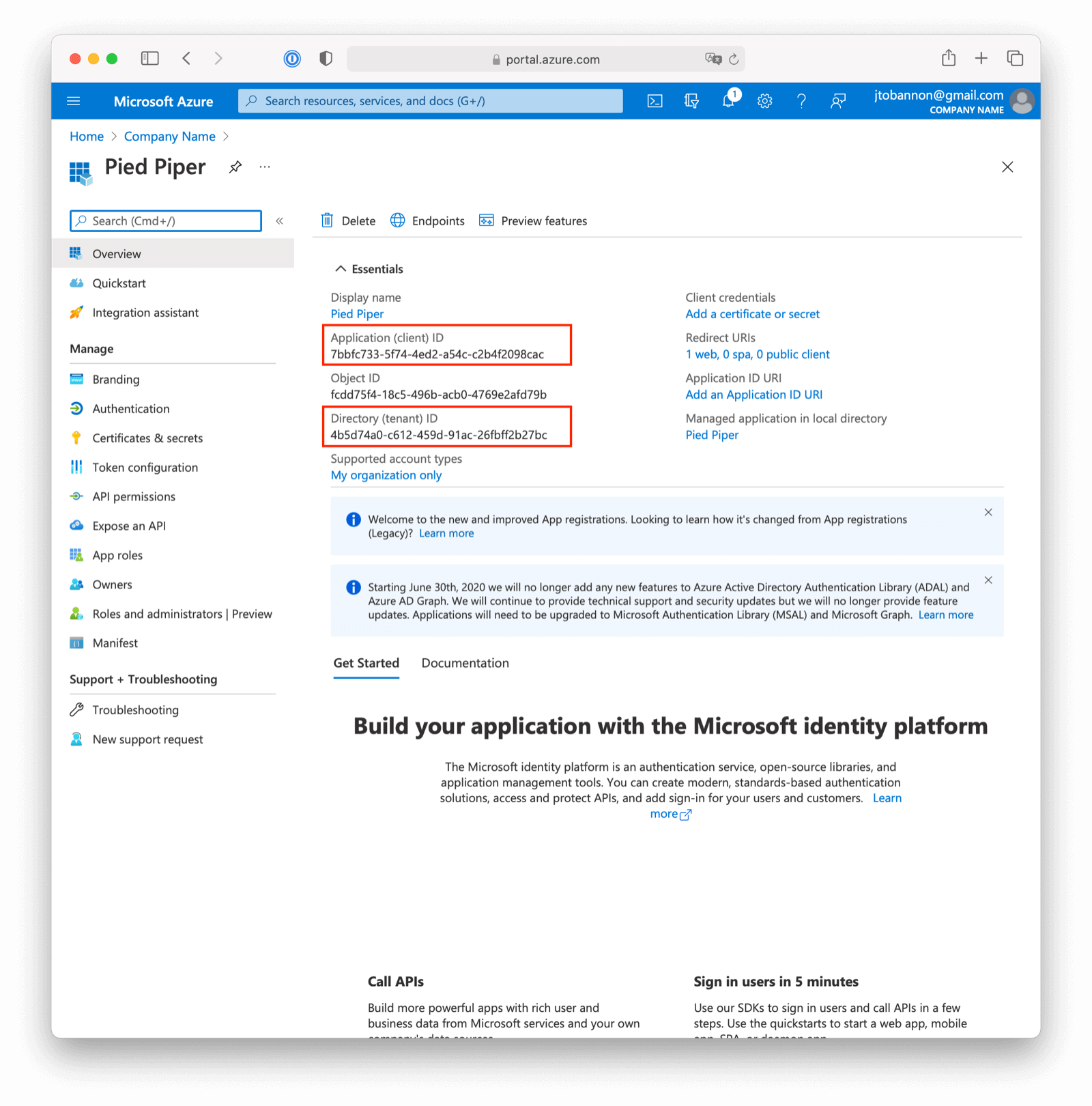The image presented is a vertical screenshot taken from a computer screen, depicting a Microsoft Azure interface. The overall design gives the impression of a box slightly lifted off the screen, with a predominantly white background.

At the very top of the screen, there is a white bar stretching across the entire width. On the upper left corner, three small circles are visible: a red circle, an orange circle, and a green circle. These are likely the window controls for closing, minimizing, or maximizing the window. Following these, several standard browser interface elements are in view, including a search bar in the center, a share icon, a new tab icon (plus sign), and options for minimizing, maximizing, or going full screen.

Below this top bar, a blue horizontal bar spans the screen with "Microsoft Azure" written in white text. Adjacent to this are more icons to the right. The user's email address and company name are displayed, alongside a small profile icon.

On the left side of the screen, a sidebar outlines navigation options. At the top of this sidebar, bold text reads "Pied Piper." Below are navigation links: Overview, Quickstart, Integration Assistant, and Manage. These options delve into further subcategories like Branding, Authentication, Certificates & Secrets. Additional options include Support + Troubleshooting, Delete, Endpoints, and Preview Features.

In the main content area, key sections are featured in the middle, marked by titles like Essentials, with descriptive content including Display Name and a welcome message. This message extends an invitation to build applications using the Microsoft Identity platform, suggesting functionalities such as calling APIs or signing in users within five minutes.